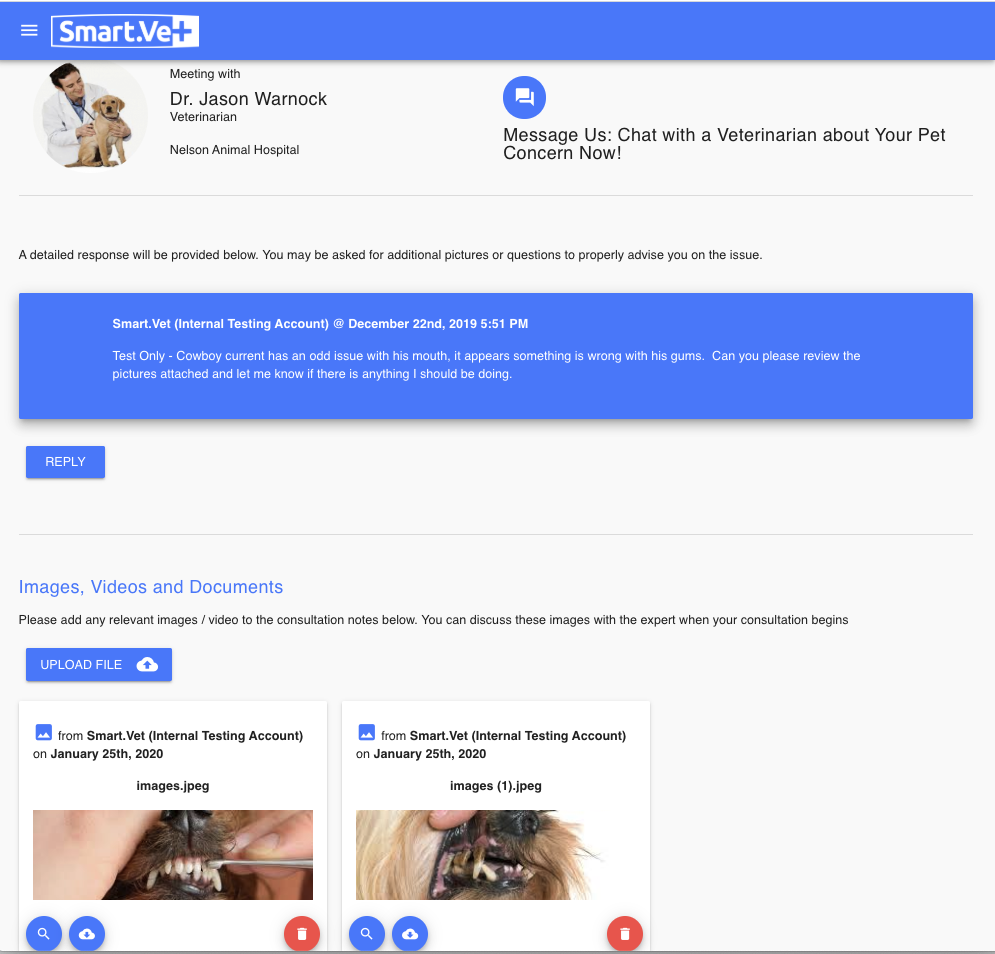Screenshot of the SmartVet Account Interface for Online Veterinary Services

In this screenshot of the SmartVet service interface, we can see several key elements that facilitate online veterinary care. At the top left corner, there is a menu button alongside the SmartVet logo, establishing the platform's branding. Below the header, the page is organized to display pertinent information about vet appointments.

The main section introduces Dr. Jason Warnock, a veterinarian associated with Nelson Animal Hospital. Accompanying Dr. Warnock's name is a thumbnail image of the doctor. Users are provided with a prompt to message Dr. Warnock, enabling real-time consultations to address immediate pet health concerns.

The appointment details reflect an interaction involving an internal testing account, dated December 22nd, 2019, specified as "test only." It mentions a pet named Cowboy, who is experiencing an issue with his gums. The note requests a review of the attached pictures to identify the problem.

Below this, the message chain is displayed, showing the history of shared images, videos, and documents pertinent to Cowboy's condition. This comprehensive layout ensures efficient communication and facilitates the proper management of the pet's health concerns through SmartVet's online service.